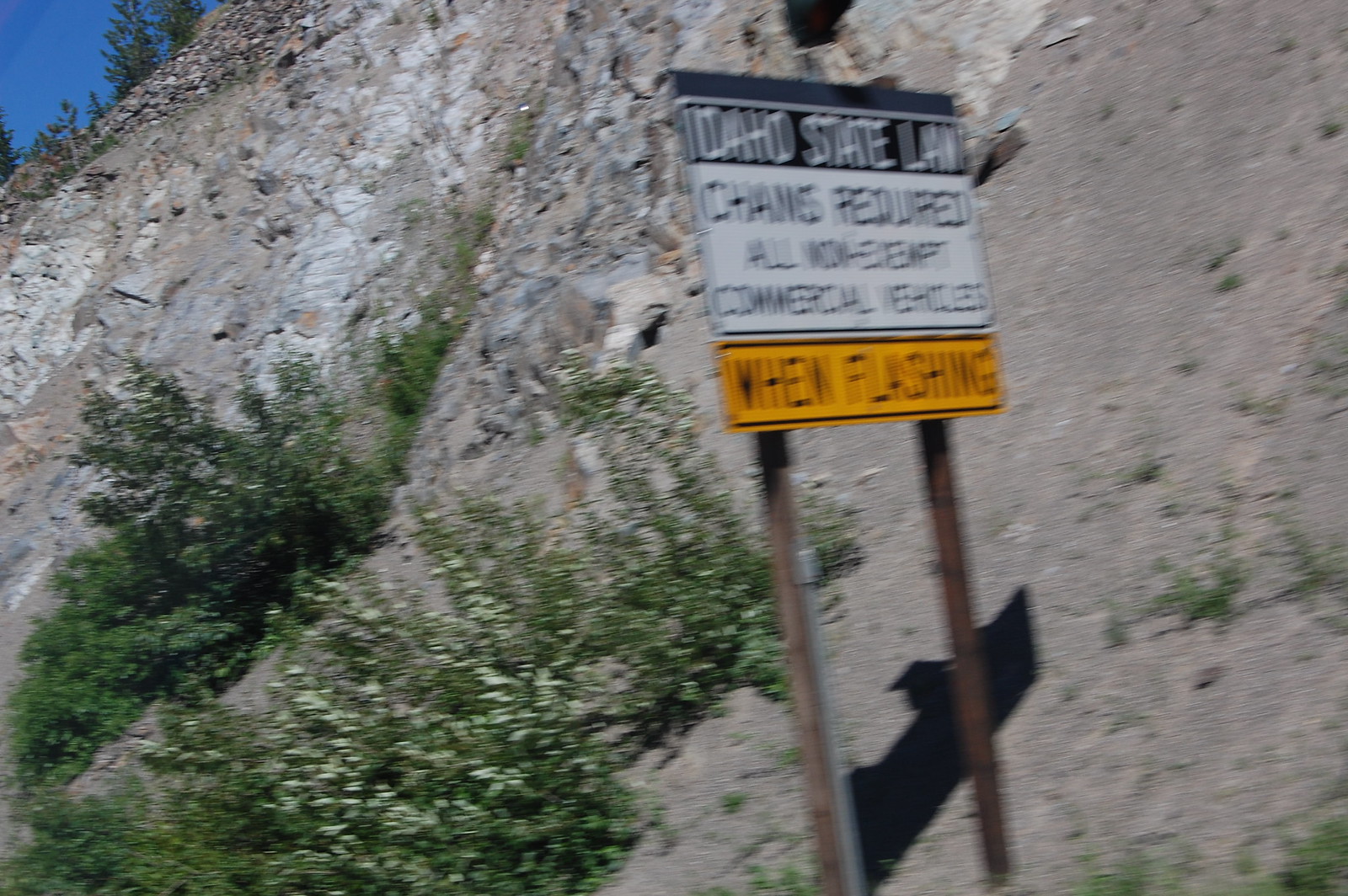This outdoor, daylight photograph showcases a steep, rocky natural stone structure composed of shades of white, gray, and brown. The cliff-like face is adorned with patches of green foliage, including noticeable bushes in the lower left and a bit of greenery in the lower right. Visible above the rocky formation are leafy green trees and a small corner of blue sky in the upper left. At the forefront, mounted on two metal posts, is a prominent sign. The top portion of the sign is white with black text reading "Idaho State Law," followed by "Chains Required" targeting all non-exempt commercial vehicles. The lower portion of the sign is yellow with black text indicating "Wind Flashing" when applicable.